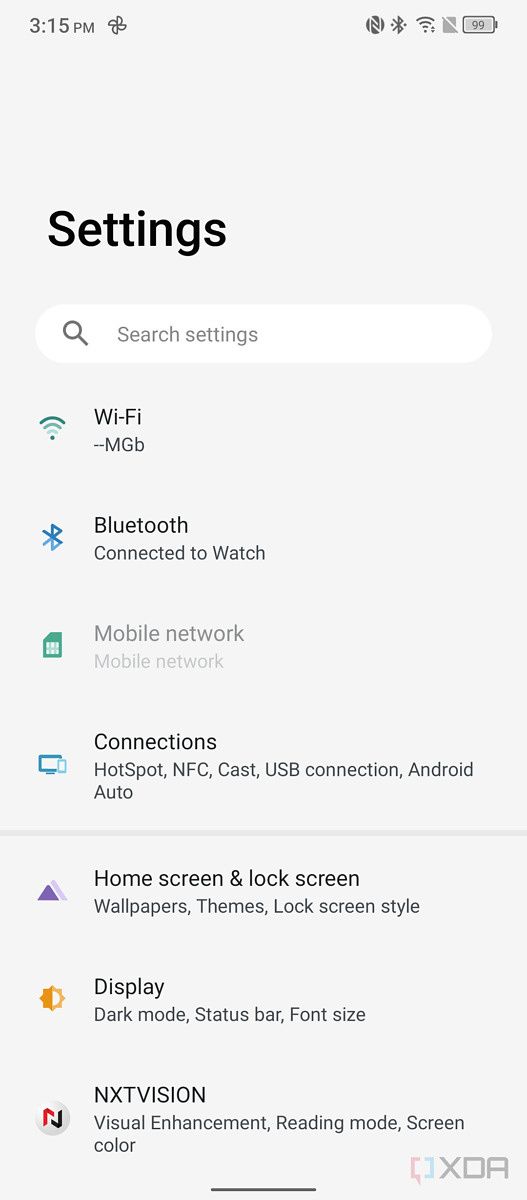### Detailed Caption for Android Phone Settings Page

This image depicts the settings page of an Android phone, characterized by a clean, user-friendly layout with a grey background. 

At the very top, the word "Settings" is displayed prominently in bold text. Directly beneath this title, there is a search bar labeled "Search settings," designed to help users quickly locate specific settings by typing keywords.

Below the search bar, several menu options are listed sequentially:
1. **Wi-Fi**: Accompanied by the familiar Wi-Fi symbol, this section allows users to toggle Wi-Fi on or off and manage connections.
2. **Bluetooth**: Marked with the iconic blue Bluetooth symbol, this option enables users to manage Bluetooth connections.
3. **Mobile Network**: This section provides information about the connected mobile network.
4. **Connections**: This menu includes additional connection options like Hotspot, USB connection, and Android Auto.
5. **Home Screen and Lock Screen**: Users can customize their wallpaper, themes, and lock screen styles here.
6. **Display**: Options within this menu include toggling dark mode, adjusting font size, and modifying the status bar display.
7. **XDR Vision**: This section allows users to enhance their visual experience, offering features like reading mode and screen color adjustments.

At the bottom right corner of the screen, the symbol "XDR" appears, possibly indicating the phone's display technology.

In the top-left corner, the current time is displayed, while the top-right corner shows the battery charge level and connection statuses, including indicators for Wi-Fi and Bluetooth.

This detailed organization and clear icons aim to aid users in navigating and customizing their device settings efficiently.